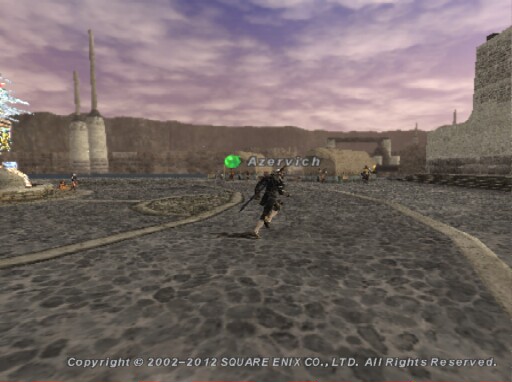This is a detailed still shot from a video game featuring the title "Azervich" prominently displayed in the center, with a green gem to the left of the text. The central figure is a character dressed in black, wearing knee-length pants and white leggings below the knee, along with black shoes. This character, seen from behind, is sprinting diagonally across a cobblestone road, with a sword strapped to his back, slightly protruding to the left side of his body.

In the distance, to the right of the character, stands a person near a doorway. The scene is framed on the far right by a cement wall. Overhead, the sky is cloudy, and the background features a flat-topped mountain range with a reddish hue. In front of this range stand two silo-like buildings with smokestacks, one noticeably shorter than the other; the shorter one's smokestack is half the height of the taller one's.

On the left edge of the image, part of a fountain is visible, displaying a design in the cement circle surrounding it. The character is positioned between two concentric circles on the cobblestone ground. At the bottom of the image, it reads: “Copyright 2002-2012 Square Enix Co Ltd. All Rights Reserved.”